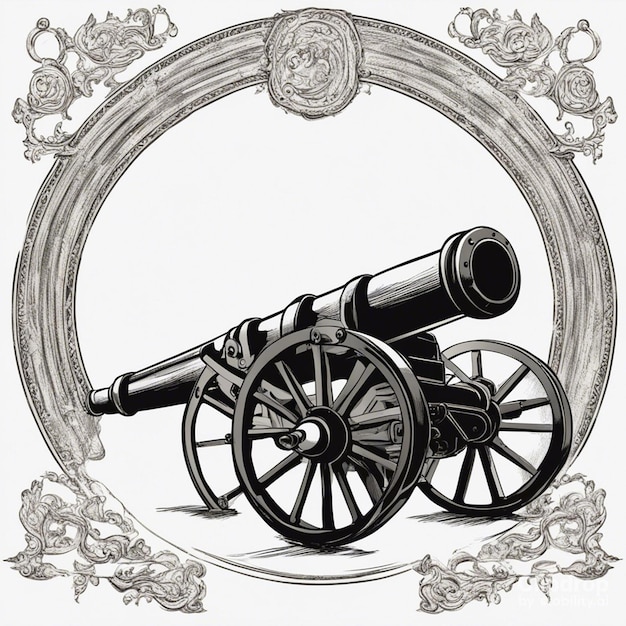The image presents a detailed, black-and-white drawing of an antique cannon, likely reminiscent of those used during the Civil or American Revolutionary War. The cannon is mounted on a sturdy base with two large wheels on either side, suggesting mobility. It also features a brace at the back end. The artwork exclusively focuses on the cannon, with no people depicted. Encircling the cannon is an ornate, spherical frame, intricately adorned with floral designs, including roses and vines, at what would be the four corners. At the top of this rounded frame, there is an indistinct medallion. The entire composition is rendered in shades of black and gray on a white background, emphasizing its artistic, old-time character.